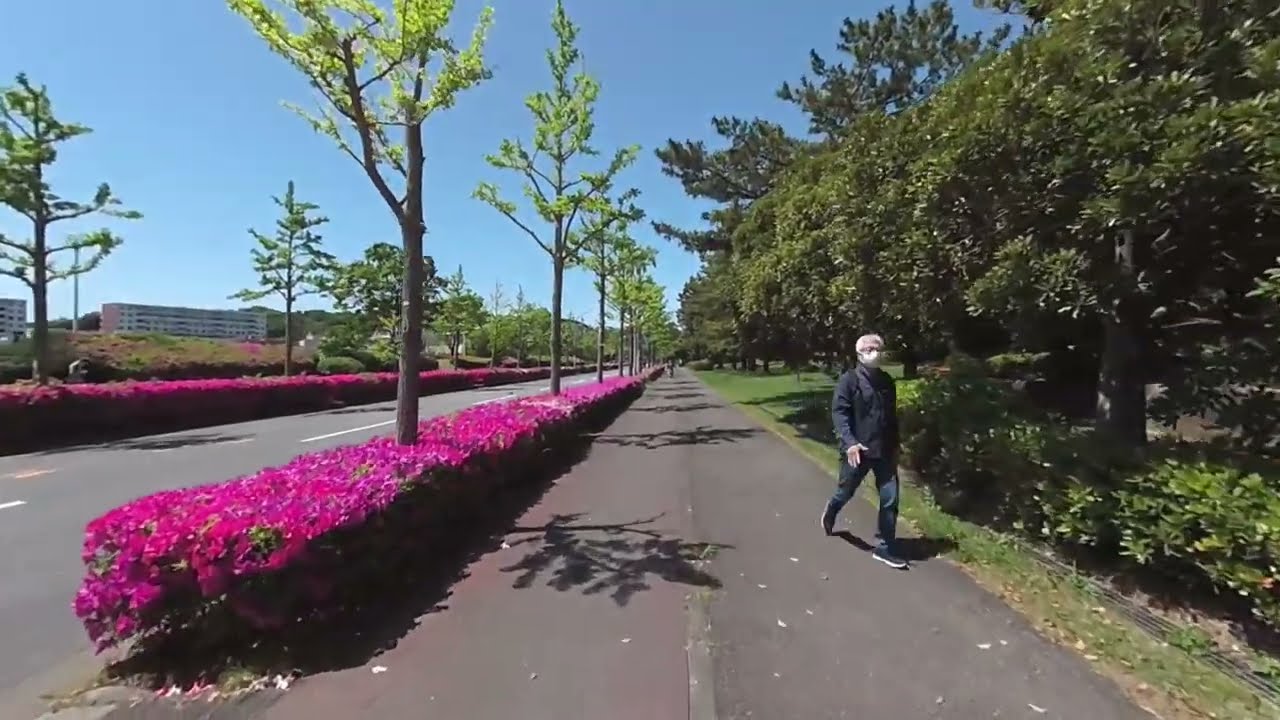In the photograph, an older man with silver hair is walking towards the camera on an asphalt-paved walking path. He is wearing a white face mask, a dark black jacket, grey pants, and running shoes. To his right, there are lush green trees and a well-maintained grassy area. On the left side of the path and extending down the center of the image, there is a median filled with fuchsia-colored azalea bushes and thin oak trees that stretch from the bottom to the top of the photo. Adjacent to this median on the left is a roadway marked with a white stripe and lined with similar pink and purple shrubberies and trees. In the background, a hillside is visible, dotted with a few prominent white buildings that are five stories high, adding urban interest to the scenic environment.